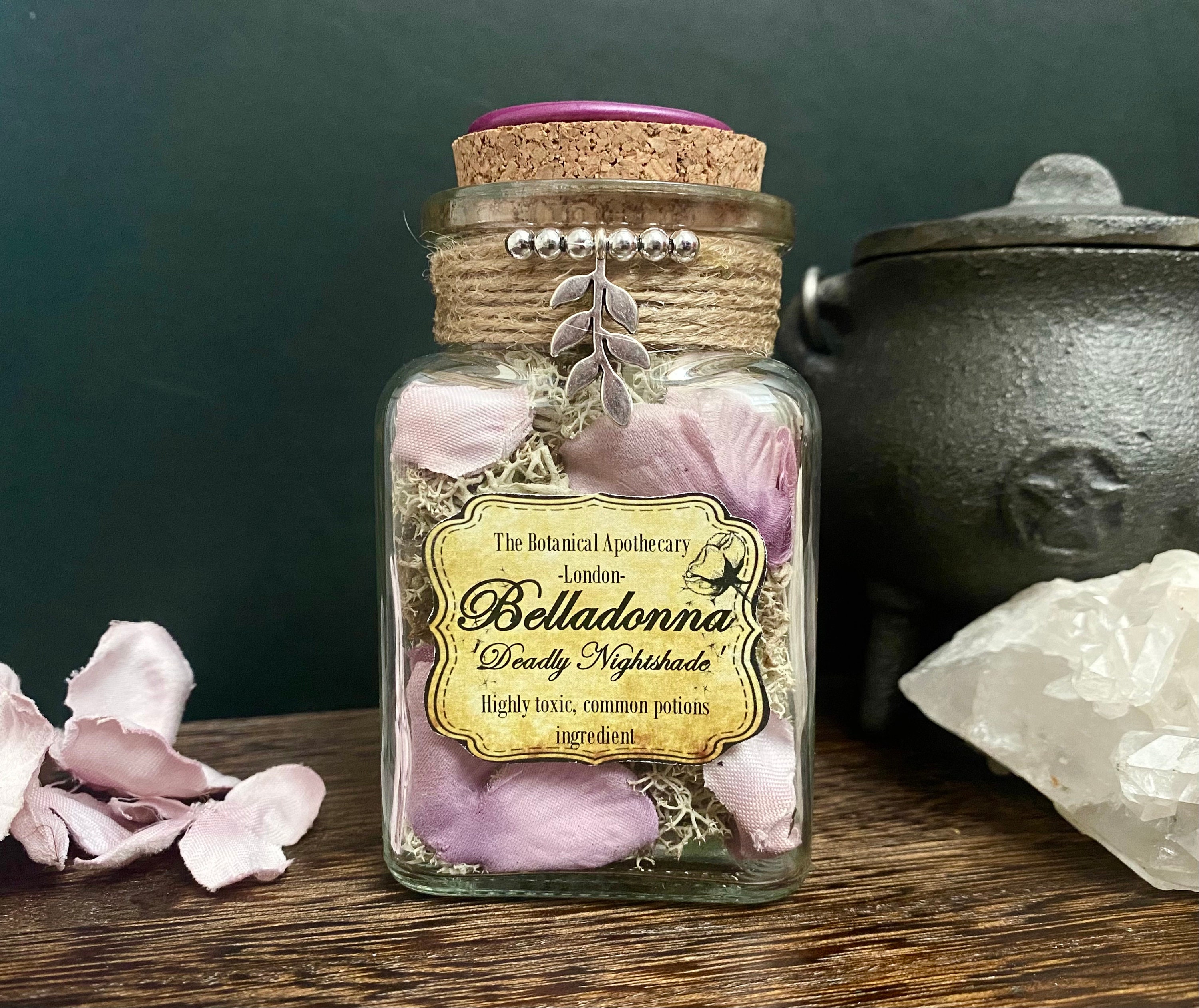In this staged photograph, a squarish bottle from The Botanical Apothecary in London, labeled "Belladonna, Deadly Nightshade, Highly Toxic, Common Potions Ingredient," sits prominently in the center. The bottle has a cork top and twine wrapped around its neck, adorned with metal embellishments resembling leaves and six small balls. Inside, the bottle appears to contain a shredded tan mixture and possibly pink petals. Positioned to the left of this central potion bottle are scattered pink flower petals, while to the right, a clear quartz crystal is seen in front of a miniature cast iron cauldron with a pentagram on its lid. The scene is set against a deep green wallpapered background, with the items resting on a wooden desk that blends darker and lighter browns. The image's color palette features shades of black, brown, lavender, purple, and white, adding to the mystical and apothecary feel of the photograph.